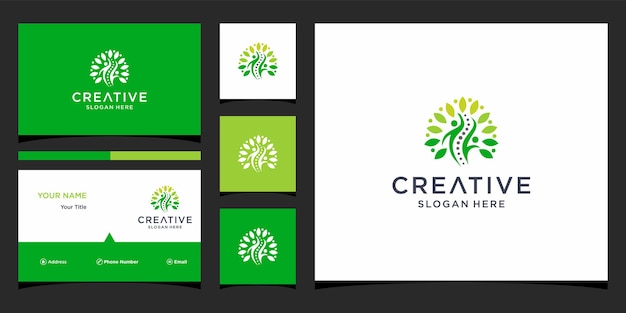The image is a rectangular, horizontal advertisement from a company that offers services to help you promote your product. The right side features a large white box with a black border, displaying the word "Creative" in large letters and "Slogan Here" in smaller text beneath it. Above "Creative" is the company's logo, which consists of a person-like figure surrounded by green leaves forming a circular pattern. 

In the center of the image, there are three smaller square boxes, each containing the same logo but with different background colors: white, light green, and dark green. On the upper left corner, there's a larger dark green box also displaying the logo, suggesting it could be a template for a business card.

On the left side, there are two areas resembling business card templates—one dark green rectangular card on top and a white card with a green base below it. The image combines multiple design elements and templates, emphasizing the company's ability to create business cards and marketing materials to promote your product effectively.